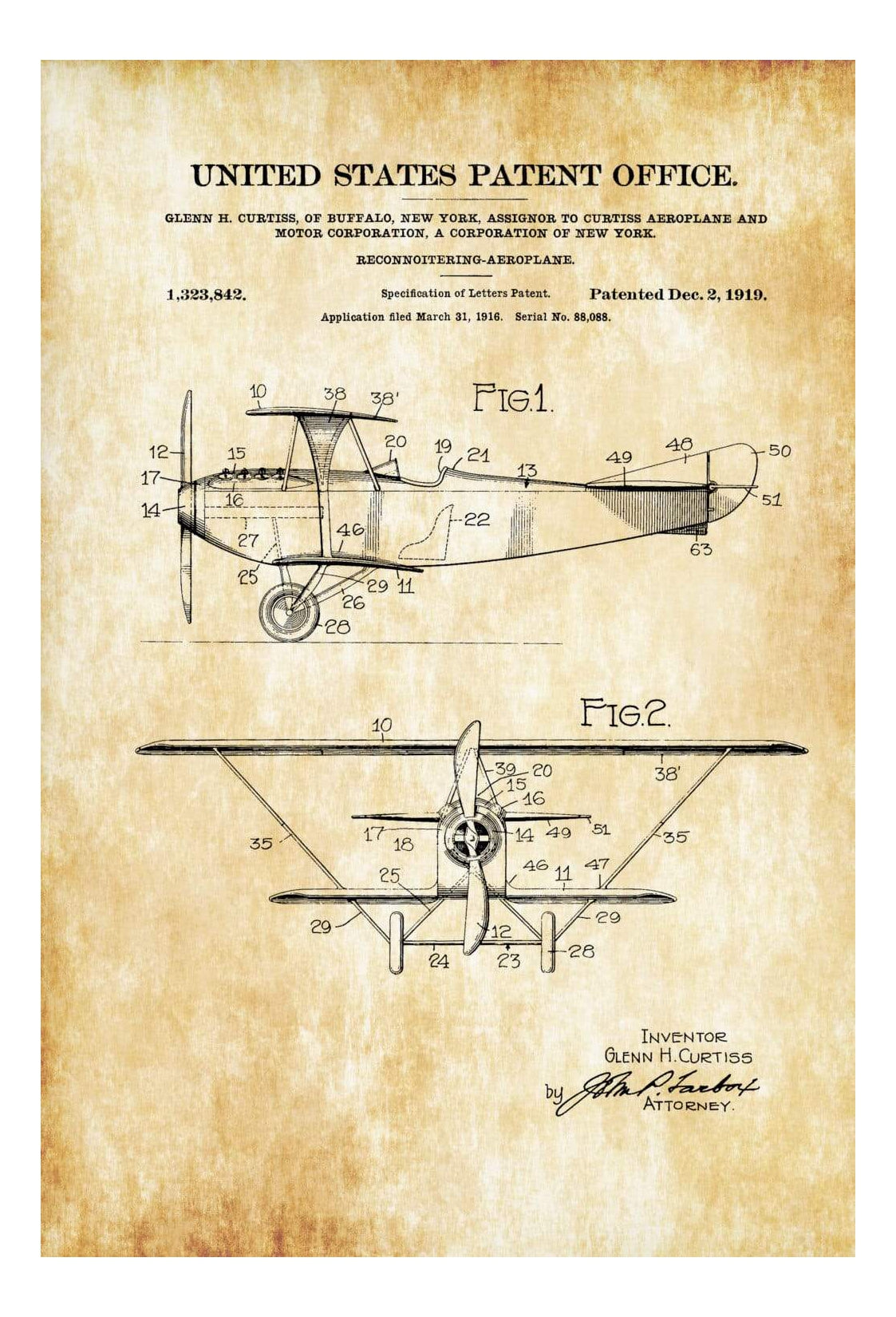This detailed antique poster displays a meticulously scanned page from the United States Patent Office, dated December 2nd, 1919. At the top of the old, brown-edged paper, it reads in bold black letters, "United States Patent Office." The inventor, Glenn H. Curtiss of Buffalo, New York, is noted as the assignor to Curtiss Aeroplane and Motor Corporation, a corporation of New York. The patent is for a "RECONNOITERING-AEROPLANE," cataloged under serial number 88,088 following an application filed on March 31st, 1916.

Centered prominently are two technical diagrams of the airplane, labeled as Figure 1 and Figure 2, each detailing various components with numbered annotations. Figure 1 presents a broadside, side-view illustration with the airplane facing left, while Figure 2 offers a top-down perspective, giving a clear view of the propeller and overall design structure. The entire document, primarily in black and white, sits on a broader orange-yellow backdrop. At the bottom, the inventor's name, Glenn H. Curtiss, is reiterated alongside the mention of an attorney, completing this historical snapshot of early aviation innovation.